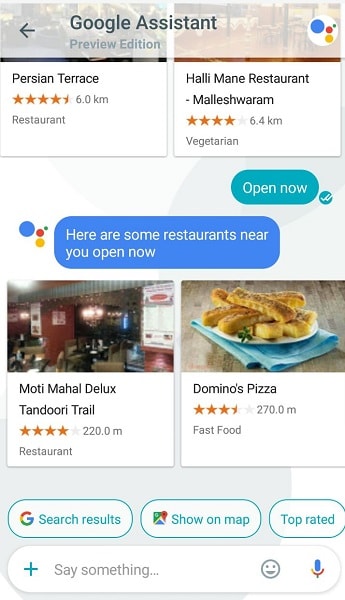The image displays a Google Assistant page. At the top, the header reads "Google Assistant" in black text, with a back button on the left and the Google Assistant icon on the right. The icon is a white circle with four smaller circles inside, colored blue, red, green, and yellow. Below the header, the text "Preview Edition" is displayed.

Further down, there are restaurant suggestions. On the bottom left, a restaurant named "Persian Terrace" is shown, rated 4.5 stars, and located 6 kilometers away. On the bottom right, a highly-rated vegetarian restaurant known for shawarma is listed, with a 4-star rating and located 6.4 kilometers away. The text "Open Now" indicates the availability status of these restaurants.

The page's background is blue and green, with white text. The conversation setup shows the user interacting with Google Assistant. The Assistant responds on the left, stating, "Here is a restaurant near you. Open now." The suggested restaurants include "Multimahal Deluxe Tandoori Trail," which is 4-star rated and 220 meters away, and "Domino's Pizza," which is 270 meters away with a 3.5-star rating in the fast-food category.

At the bottom, there are buttons labeled "Search result," "Show on map," and "Top rated." Additionally, there is a text input box where users can type their queries or responses.